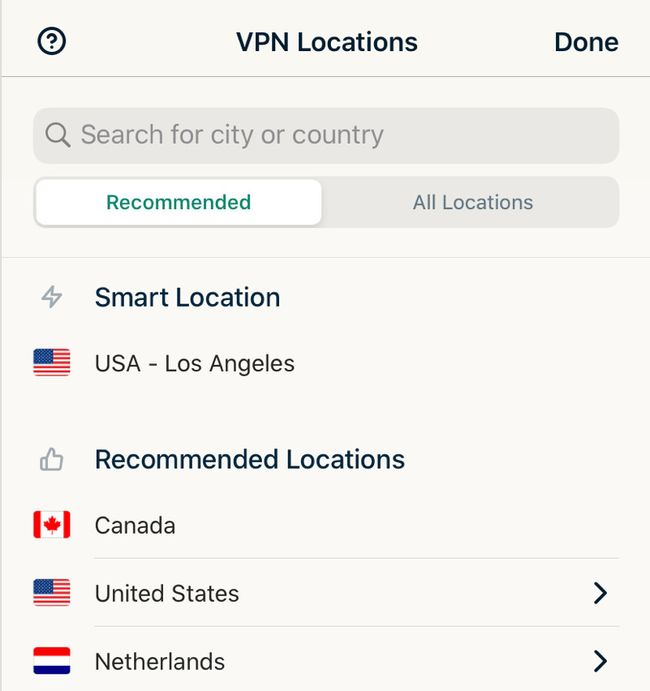A screenshot of a mobile phone displays the UI of a VPN application. At the top left, there is a question mark icon, followed by the title "VPN Locations" in bold black text, with a "Done" button to the right, also in bold black font. Below this header, a gray search box prompts users to "Search for city or country." Beneath the search box, two tabs are present: "Recommended," highlighted with a white background, and "All Locations," set against a gray background. 

Further down, the text "Smart Location" appears in bold blue font, accompanied by a U.S. flag icon and labeled "USA - Los Angeles." Adjacent to these labels is an inactive thumbs-up icon. Below this section, the text "Recommended Locations" is displayed in blue bold font, followed by a list of countries with their respective flags: Canada (without an arrow), the United States (with a right-pointing arrow), and the Netherlands (with a right-pointing arrow). The entire interface is set against a white background for clarity.